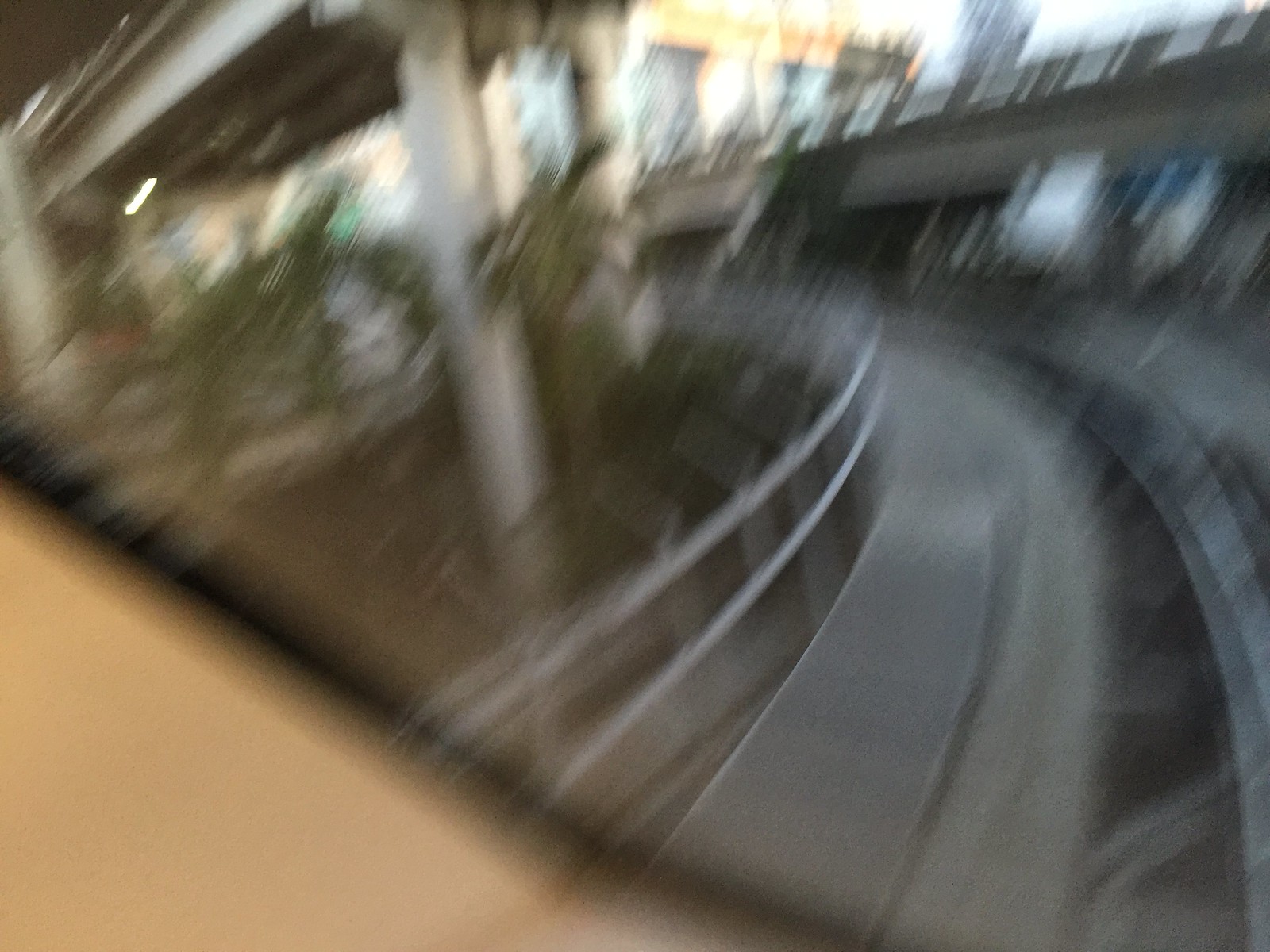This photograph, taken from inside a vehicle, is extremely blurred and out of focus. The scene is set outside in daylight, with sunlight shining on the various elements. Dominating the lower left portion of the image is a beige, triangular section, suggesting the interior reflection from the vehicle. To the lower right, a road curves leftward, bordered by a guardrail. The upper left corner reveals an overpass, while the upper right corner presents another separate roadway. The background showcases a building with tall, rectangular, glass windows framed by beige and orange walls. Scattered throughout the scene are concrete supports and some foliage, possibly palm trees. The overall image exudes a chaotic mix of urban infrastructure, with shades of gray illustrating various walkways or driveways.